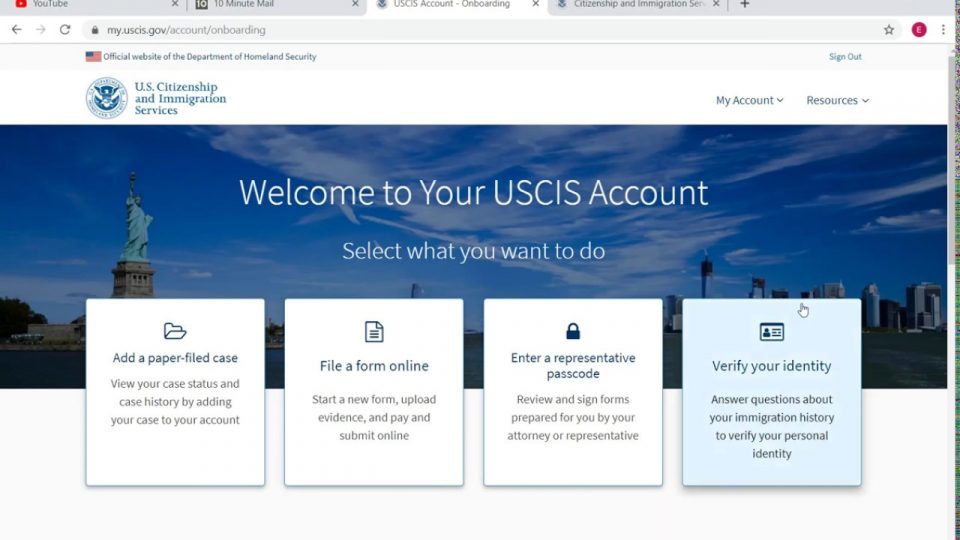The image displays a webpage from the official U.S. Citizenship and Immigration Services (USCIS) website, specifically the onboarding section at my.uscis.gov/account/onboarding. The browser window containing this page is not visible, but it is noted that there are four tabs open.

The website features the emblem of the Department of Homeland Security, and the interface includes options such as "My Account," several resource pull-down menus, and a "Sign Out" button. The main content greets the user with, "Welcome to your USCIS account, select what you want to do."

The background features an image of the Statue of Liberty with the New York City skyline against a blue sky with scattered clouds. Superimposed on this background, there are four interactive boxes:

1. **Add Paper-Filled Case**: Allows users to view their case status and case history by adding their case to their account.
2. **File a Form Online**: Users can start a new form, upload evidence, and complete payment and submission online.
3. **Enter a Representative Password**: Enables users to review and sign forms prepared by their attorney or representative.
4. **Verify Your Identity**: Users can answer questions about their immigration history and verify their personal identity.